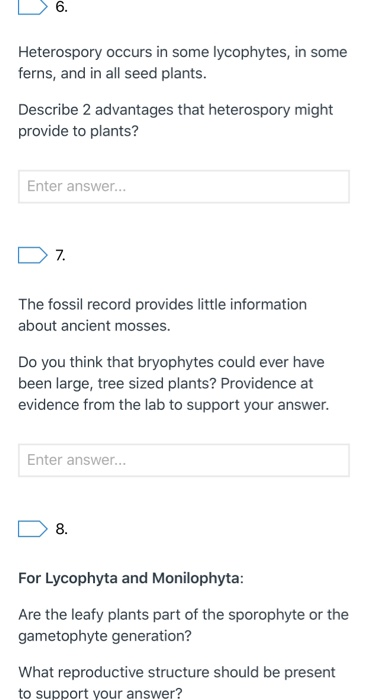The image presents three paragraphs from an examination paper focused on genetics in plants, as well as the fossil records of ancient mosses, lycophytes, and monilophytes. The questions, numbered 6, 7, and 8, appear to be part of a botany exam, with dedicated spaces provided for students to write their answers. The content suggests an in-depth assessment of students' understanding of plant evolution and genetic characteristics.